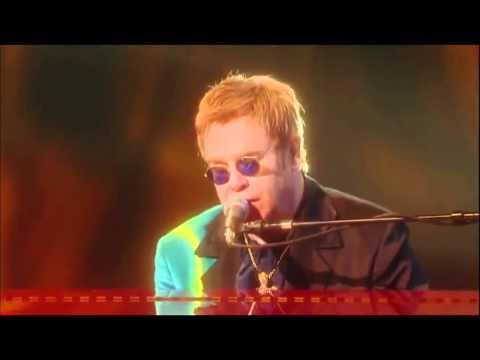The image depicts a vibrant color photograph of a television screen showing the iconic singer Elton John. Positioned in the center, Elton John sports his signature short hair, dyed a striking blondish-orange hue. His distinctive style is further accentuated by round sunglasses with purple lenses, adding a touch of mystery and flair to his appearance. Elton John is clad in a sharp black suit that features a unique turquoise section on the left side, injecting a pop of color into his ensemble.

He appears to be performing, as indicated by the microphone held on a stand, with the microphone handle extending off the right edge of the image. His posture suggests he is seated while singing, immersed in his vocal performance. Below Elton John, there is a red bar, possibly part of the TV broadcast graphics or subtitles.

The background is intentionally blurred, ensuring all focus remains on Elton John. Additionally, the image is framed by thick black horizontal lines at both the top and bottom, giving it a cinematic appearance. The attention to detail in this photograph captures not just the essence of Elton John's performance but also the atmosphere of the scene.